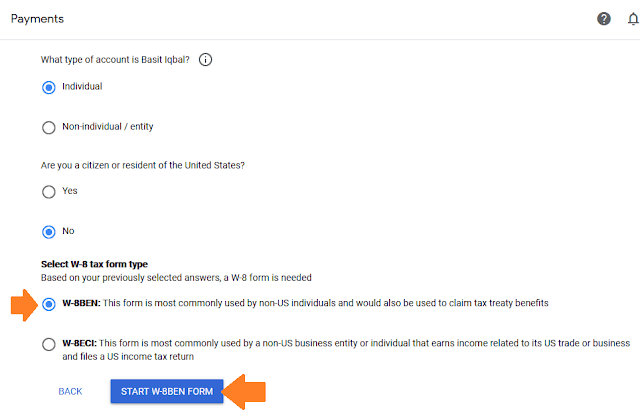The image has a clean white background with the heading "Payments" displayed at the top in black font. To the right of this heading, there is a gray circle containing a white question mark, and a gray bell icon outlined in gray. Beneath this heading, a long horizontal line spans the width of the image. 

Below the horizontal line, a small black font text asks, "What type of account is this?" with an additional possibly saying "Basal" followed by "IQ BAL?" with a gray circle featuring a small "i" icon next to it.

Further down, there are two account-type choices: "Individual" and "Non-individual/Entity." Each option is preceded by a circle; the one next to "Individual" is filled with turquoise, indicating it is selected, while the "Non-individual/Entity" circle is empty.

The next question, "Are you a citizen of the United States?" presents two options: "Yes" and "No," with the "No" option highlighted in turquoise.

Following this, there is a bold black header that reads, "Select W-8 Tax Form Type." Underneath, in regular black font, it explains: "Based on your previously selected answers, a W-8 form is needed." Below this text, there are two bullet points, the first of which is colored in turquoise and positioned to the left of a bold yellow and orange arrow pointing right. This section also contains the bolded black text in capital letters "W-8BEN:" followed by the explanation: "This form is most commonly used by non-US individuals and would also be used to claim tax treaty benefits."

The second bullet point is not highlighted, and the bold text reads, "W-8ECI," with the explanation: "This form is most commonly used by a non-US business entity or individual that earns income related to its US trade or business and files a US income tax return."

At the bottom of the image, the word "BACK" is displayed in all capital turquoise letters, accompanied by a blue horizontal rectangle with the words "START W-8BEN FORM" in white capital letters. A larger orange arrow points toward the form to the left.